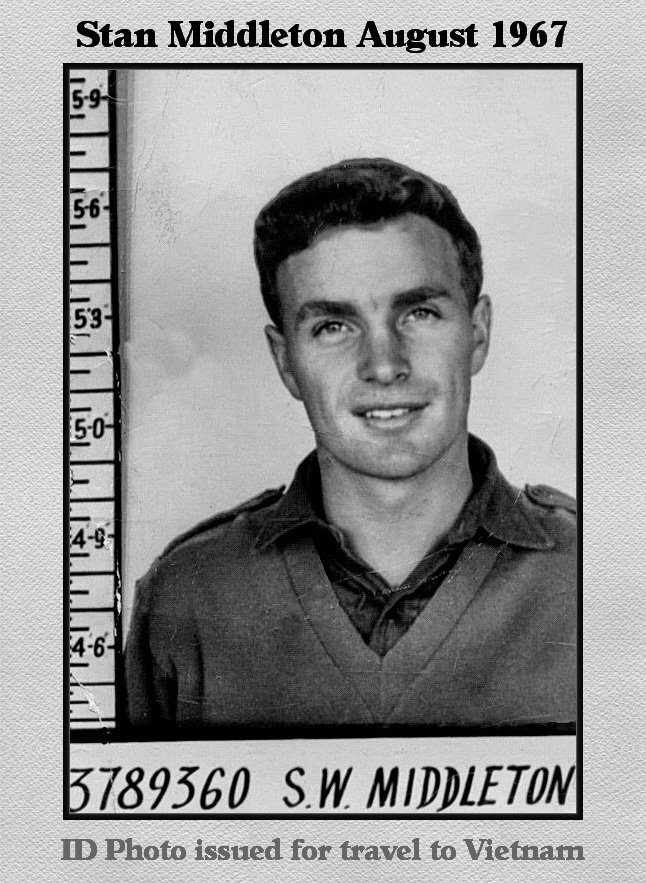The image features a vintage ID photo from August 1967, set against a multicolored gray background with various shades of gray, black, and white. The ID photo, positioned centrally within a black-bordered portrait box, depicts a young clean-shaven man with dark hair, wearing a collared shirt under a V-neck sweater. The man, identified as Stan Middleton, is shown smiling slightly and looking directly at the camera. To the left of his image, there is a measuring stick indicating his height at about 5’7”. At the top of the image, the text reads "Stan Middleton, August 1967, 3789360SW Middleton, ID photo issued for travel to Vietnam," denoting its purpose as an ID photo for travel.